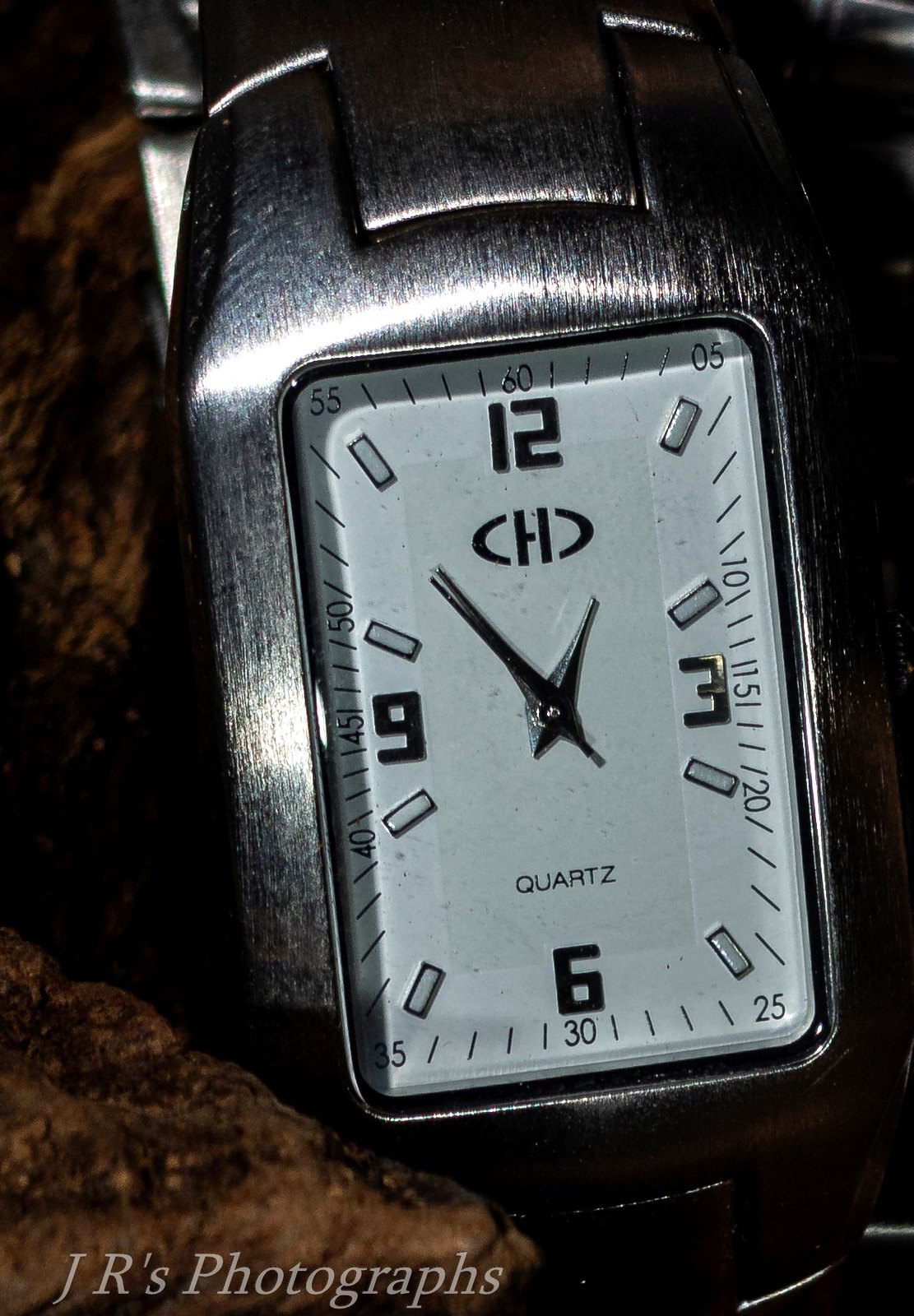The image is a close-up of a rectangular, silver wristwatch with a light grey analog face. This timepiece prominently displays the numbers 12, 3, 6, and 9, with slender rectangular markers at the other hour positions, all pointing radially inward. The word "Quartz" is visible on the watch face, indicating its movement type. In the bottom left-hand corner of the watch face, the text "JR's Photographs" is etched, suggesting it's either a brand or the photographer's watermark. The background features a distinctive logo comprising the letters "C," "H," and a reversed "C," although their specific arrangement is not entirely clear. The watch appears to be positioned on a surface with dark and slightly brownish tones, alongside black, rock-like elements.